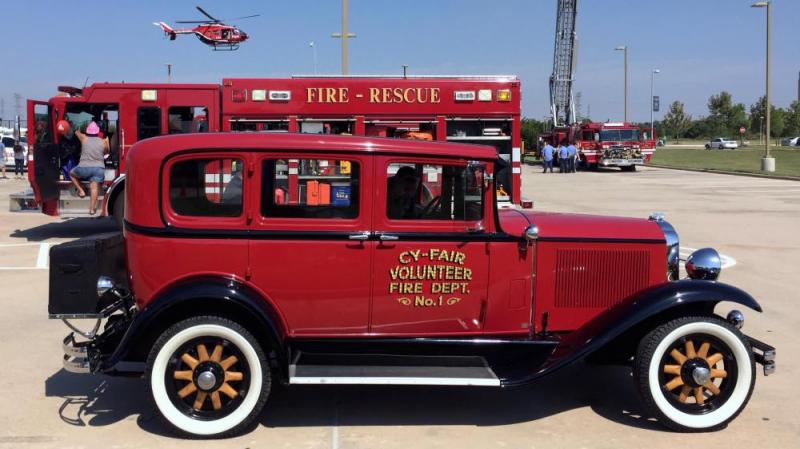The rectangular, landscape-oriented color photograph captures an outdoor scene in a spacious parking lot under a clear blue sky. The focal point is a striking display of fire trucks from various eras, suggesting a possible show or exhibition. In the foreground, a vintage Model T Ford fire truck draws immediate attention. This two-door coupe, featuring suicide doors that open opposite to traffic, is painted in vibrant red with black accents and a black stripe running its length. The truck boasts polished chrome headlights positioned on little bars over its black fenders, oversized whitewall tires with beige spoke wheels, and a box on a support bracket at the back. Its highly polished radiator gleams under the sun. On the front passenger side door, the gold text with a black shadow reads "PSY-FAIR, Volunteer Fire Department Number 1."

Behind this vintage beauty stands a more modern fire rescue truck, similarly red, bearing the label "Fire and Rescue." Stretching into the upper right corner, a contemporary fire truck with an extendable ladder poised skyward sits, surrounded by several firefighters in light blue tops and dark blue bottoms, exemplifying the dedication and readiness of modern emergency services. 

In the top left, a red and black helicopter hovers, perhaps used for aerial spotting, adding an element of dynamic action to the scene. The backdrop of the image features a red building with several open bays and the sign "FIRE-RESCUE" in gold letters, emphasizing the setting as a hub of firefighting activity. The entire composition blends the historical with the contemporary, celebrating both the past and present of fire rescue services.